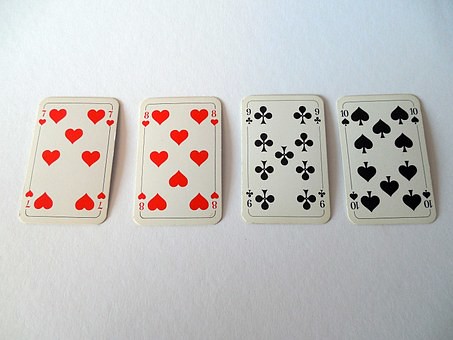This color photograph features a detailed arrangement of four vintage playing cards, carefully laid out in a single file line on a pristine white surface. Each card showcases a distinct suite and number, giving a rich glimpse into the craftsmanship of antique card design. 

From left to right, the cards are as follows: 
1. The seven of hearts, which displays small, bright red number sevens in each corner and seven vivid red hearts in the center.
2. The eight of hearts, adorned with tiny eights in all corners and eight red hearts neatly positioned in the middle.
3. The nine of clubs, showing a black number nine in each corner and nine black clubs spread across the center.
4. The ten of spades, featuring black number tens in every corner and ten black spades arranged in the middle.

The cards’ beige backgrounds and rounded corners contribute to their vintage aesthetic, standing out sharply against the immaculate white background that holds no other markings or writing. This image captures the timeless elegance and intricate design of classic playing cards.